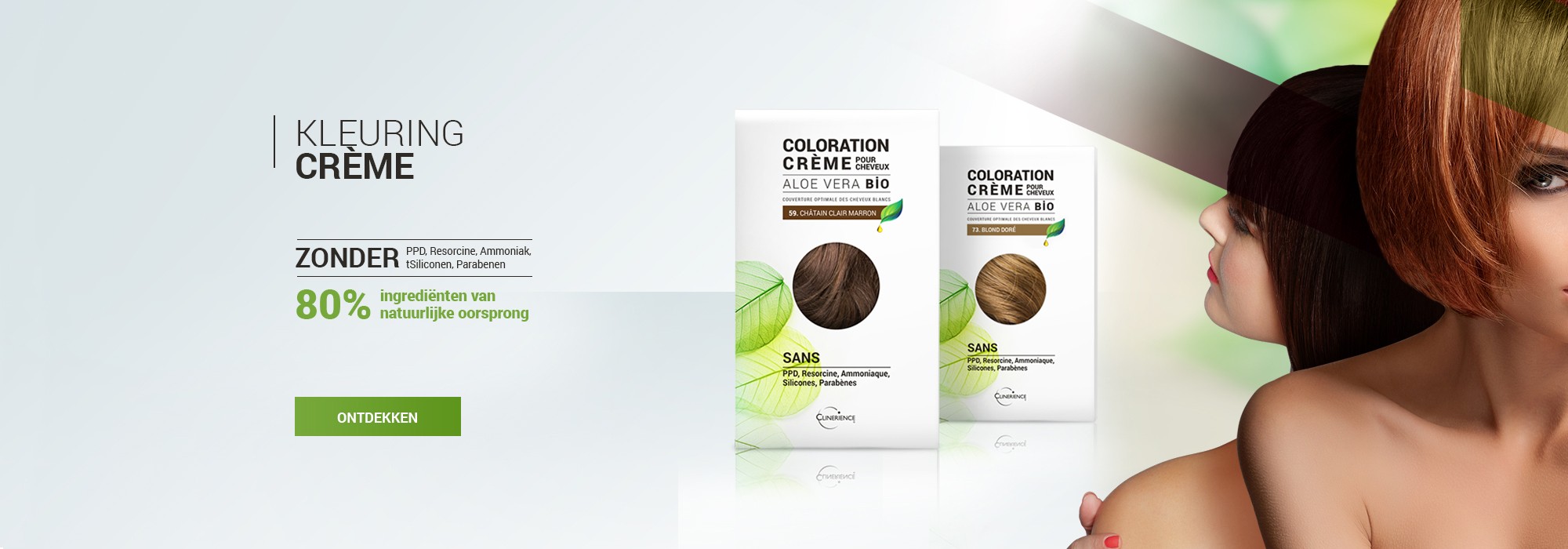This advertisement for Coloration Cream uses a predominantly off-white color palette. Located slightly left of center, the text "Clearing Cream" is printed in bold black font. Below this, it states "Zander," followed by smaller, unreadable text, and then "80% Ingredienten van Natuurlijk Oorsprong" in green, which translates from Dutch as "80% Ingredients of Natural Origin." Beneath this is a green bar with illegible white writing.

At the center of the image, there are packages of the Coloration Cream hair dye. The top of the box reads "Coloration Cream" in black, and "Aloe Vera Bio" in smaller text below. Each package features a circular window showcasing close-up images of hair: the left displays a brunette shade labeled "Chaton Claire Marron" and the right a dirty blonde shade labeled "Blonde Doré." More black text is visible below these images. To the left of each box, a leaf graphic is displayed: green for the top package and yellow for the bottom.

On the right side of the ad, images of two animated women are visible, only showing half their faces. They pose back to back, each with different hair colors. The text further emphasizes the natural and chemical-free components of the product, listing "Sans PPD, Ammoniac, Silicone, Paraben" (without PPD, ammonia, silicone, and parabens).